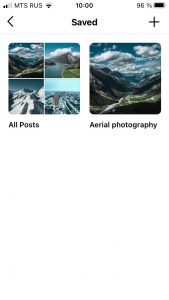This blurry screenshot captures a section of a mobile application, potentially a gallery or profile showcasing various options. The upper part of the screen displays typical phone settings, including a cellular signal strength indicator followed by the letters "MTS RUS," a Wi-Fi signal strength meter, the current time centered, and a battery icon showing 96% next to the battery percentage. 

The visible interface appears to be a menu labeled "Saved," indicating saved items, with a back arrow on the left and a plus symbol, likely for adding new content, on the right. Below this title, two distinct thumbnail icons are visible. The first thumbnail, labeled "All Posts," is a collage of four different images, suggesting it contains multiple pictures within the gallery. The second thumbnail features an image of mountain ranges with clouds in the background and is labeled "Aerial Photography."